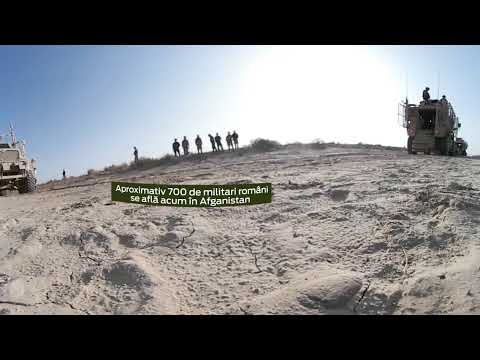The photograph depicts a military scene in a desert landscape, specifically in Afghanistan. In the foreground, there is a hill covered in sand and dirt that rises towards the background. At the top of the hill, several soldiers stand in a line, appearing to observe the surroundings. Centered in the middle of the image is a banner with text in a foreign language, which includes the words "approximately 700," "military," "Romania," "Afla," "Akum," and "Afghanistan." On the left side of the hill, a military jeep is visible, while on the right side, a larger tank-like vehicle can be seen with a man standing on top of it. The scene is brightly lit by the sun, and the sky is a clear, vibrant blue. The overall impression is that of a strategic military position in the rugged terrain of Afghanistan.